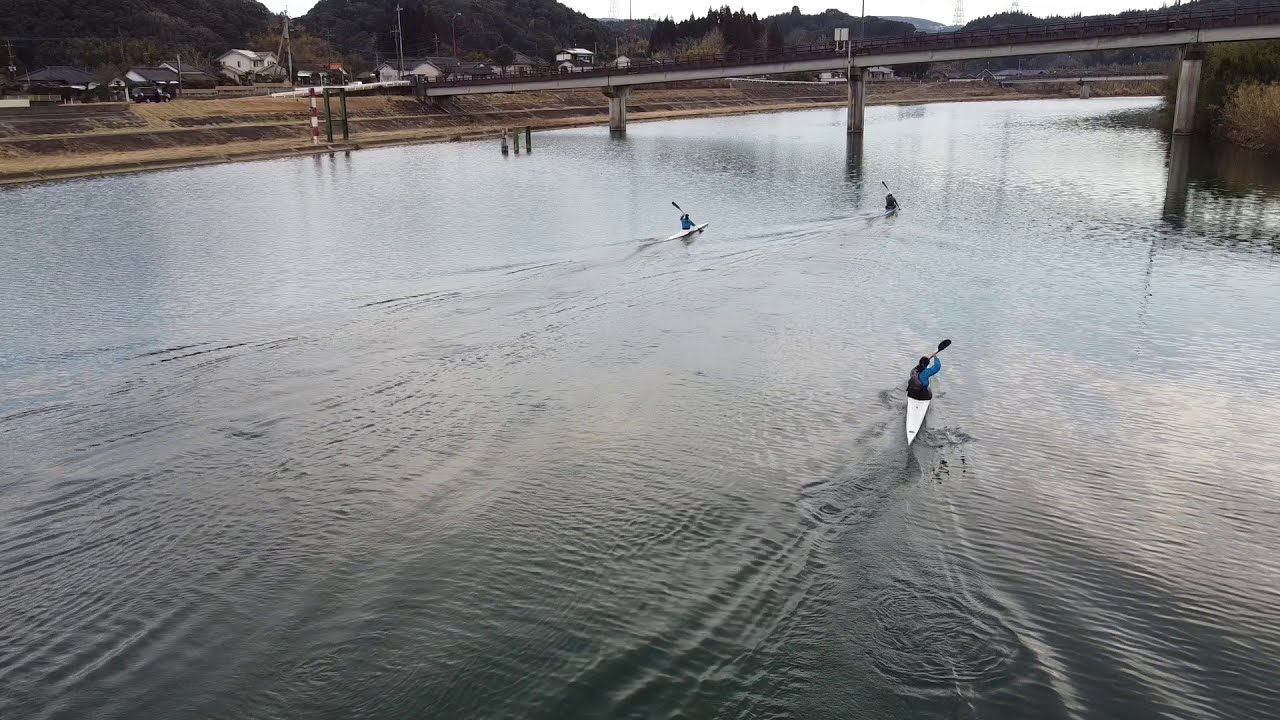The image is a detailed color photograph taken from an aerial perspective, showcasing a group of three kayakers paddling down a river. Each kayaker, positioned in a sleek, narrow white kayak, is seen holding a double-ended black paddle. The scene is set on a relatively overcast day, casting a reflection of the gray sky on the dark, rippled water, which is fairly rough, indicating a likely presence of wind. The water, covering the majority of the image, is interspersed with visible wakes and currents created by the movement of the kayaks.

The kayaker closest to the viewer is distinguishable by their light blue attire, while it is noted that the kayaker to the left in the distance also appears to be wearing blue, whereas the farthest kayaker's clothing is indeterminable, likely darker. In the midground, an overhead bridge or overpass, supported by three pillars, spans across the river, providing a sense of depth and perspective as the kayakers move towards it.

Positioned on the left bank of the river are several structures, including houses and various buildings, nestled along rocky hills. Behind these structures are tall, dark green trees that stretch into the background, where another bridge is faintly visible, further emphasizing the expansive and scenic nature of the setting.